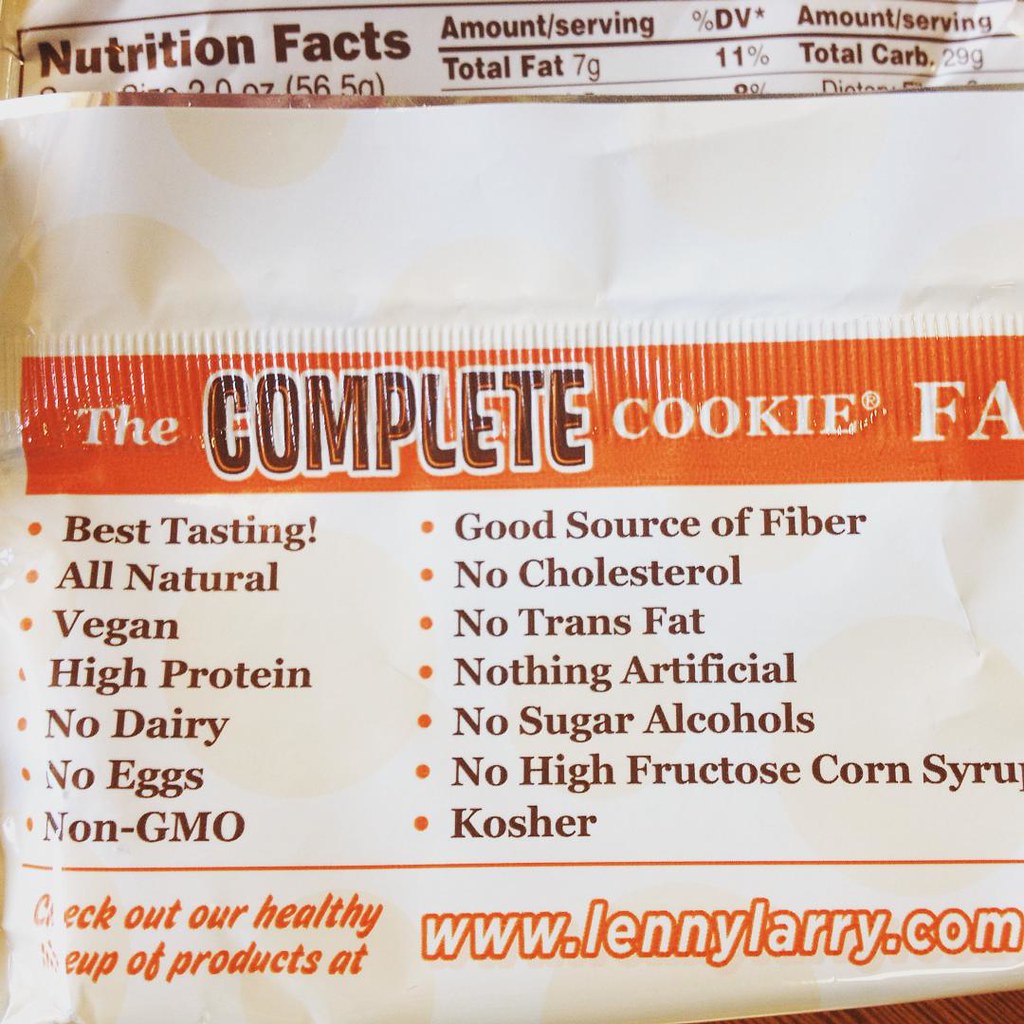This image depicts the folded packaging of a cookie product against a white background. The visible portion displays several sections of the packaging's nutrition and product information. At the top, a section of the nutrition facts is just barely visible, showing "Amount/Serving" with "Total Fat 7 grams" and "Total Carbs 29 grams," the rest concealed by the fold.

Below this, a horizontal orange band spans the width of the packaging, adorned with the phrase "The Complete Cookie" in bold lettering. The text "fa" is partially cut off, hinting at additional words beneath the fold.

To the right, a column lists product attributes in brown lettering, each prefaced by little orange bullets. This column highlights key features: "Best Tasting, All Natural, Vegan, High Protein, No Dairy, No Eggs, Non-GMO, Good Source of Fiber, No Cholesterol, No Trans Fat, Nothing Artificial, No Sugar Alcohols, No High Fructose Corn Syrup, and Kosher."

An orange line separates this information from a smaller section below, where a message invites consumers to "Check out our healthy variety of products at www.lennylarry.com."